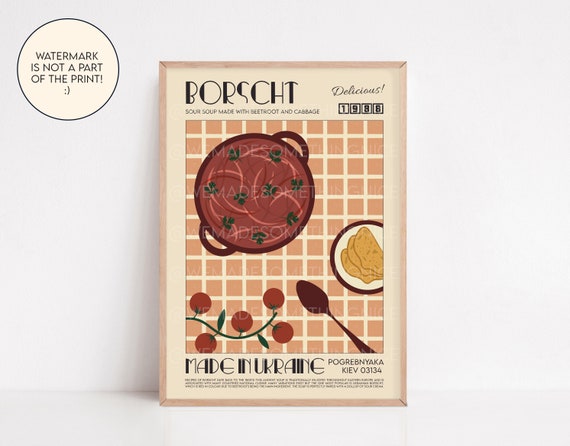The photograph is rectangular and features a framed poster leaning against a white wall, resting on a white surface. The wooden-framed poster has a light beige or off-white backdrop and prominently displays the word "Borscht" in bold, Art Deco style text at the top left, with the word "Delicious" in thin black cursive at the top right. Underneath, in a refined black typeface, are the words "Sour Soup made with beetroot and cabbage," followed by the date "1988".

Central to the poster is an illustration depicting a burgundy pot filled with red soup garnished with green leaves. The pot, equipped with two handles, sits on a pink and white cross-hatched tablecloth. Nearby, a small plate holds bread-like objects, and scattered around are red tomatoes on a green vine and likely smaller tomatoes, enhancing the food motif. At the bottom, the text "Made in Ukraine" appears in a stylized manner, accompanied by some smaller, unrecognizable text and the number "03134".

A conspicuous detail in the top-left corner of the poster is a circle with a black outline and white center that states, "watermark is not part of the print."